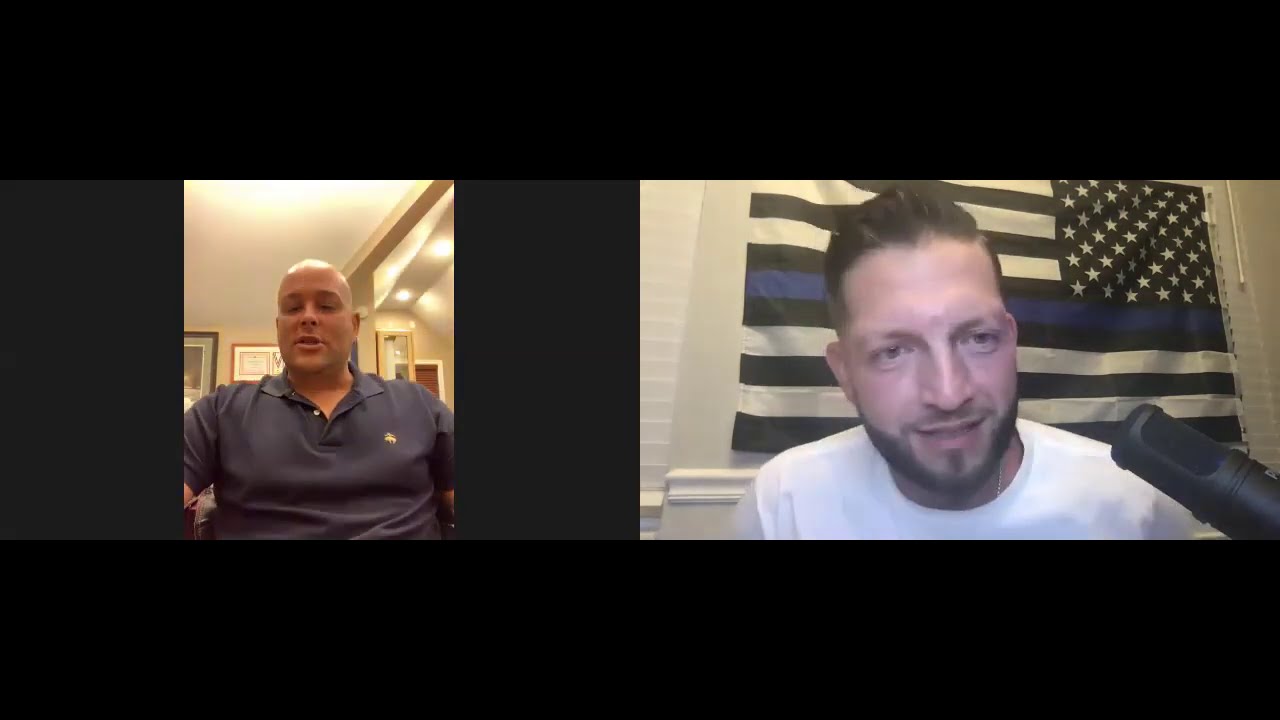The image appears to be a screen grab from a live stream featuring a split-screen conversation between two men. The man on the left, who is bald, is wearing what seems to be a navy polo shirt with a yellow logo, possibly a Ralph Lauren shirt, sitting in front of a living room-like setting. Behind him, there are framed photos and visible ceiling lights, indicating he is indoors. To his right, there is an open doorway or hallway. The man on the right, who looks to be in his 30s with greased-back black hair, is sporting a beard and mustache. He is dressed in a white t-shirt and has a microphone placed in front of his face. Behind him is a "thin blue line" American flag, which is mostly black and white with a single blue stripe, often associated with conservative politics.